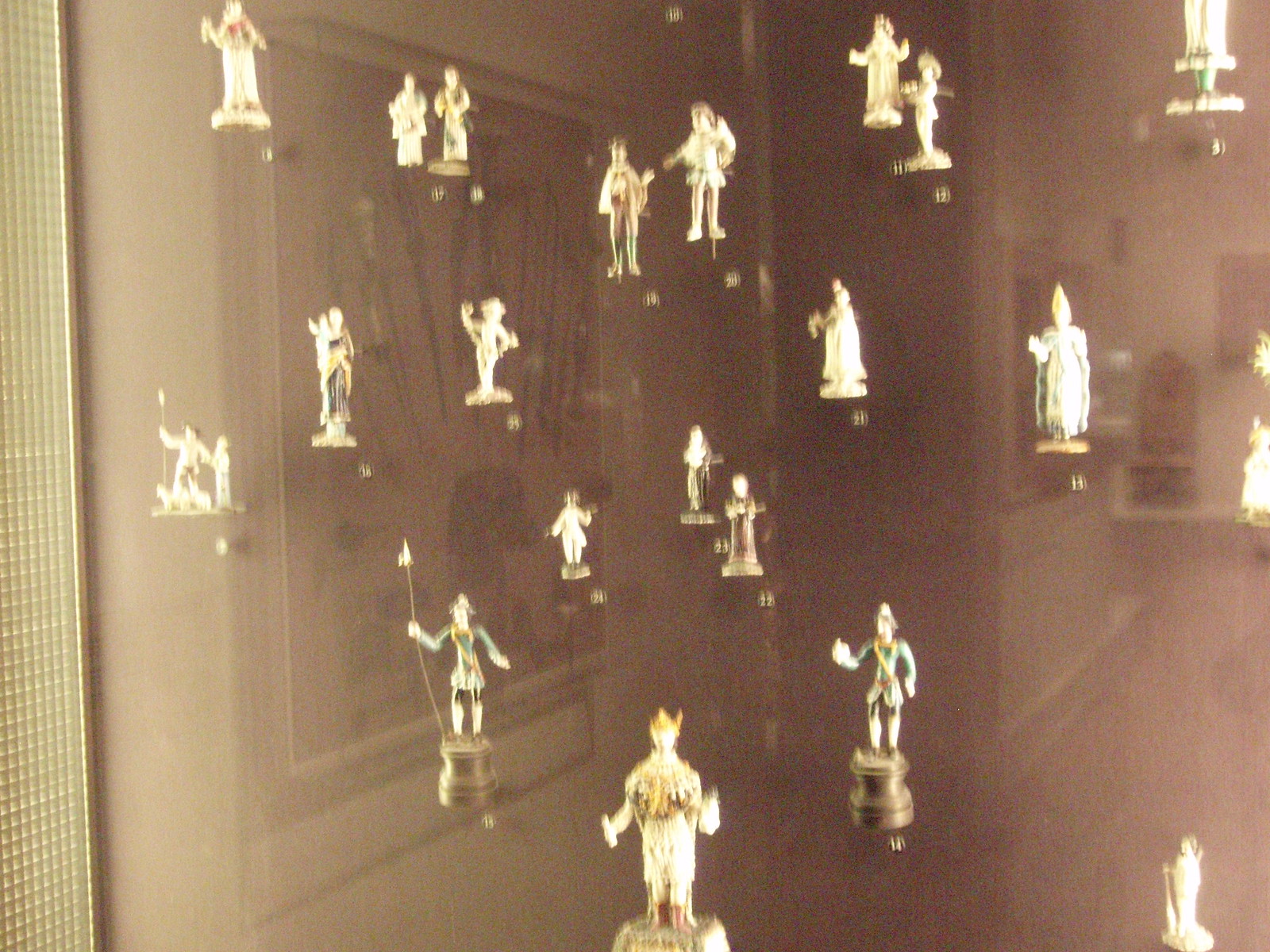The image depicts a detailed and visually complex display, primarily characterized by a black background with numerous light-colored pegs arranged randomly. Atop these pegs are a diverse array of small figurines, ranging from miniature to medium action figure size, including representations of soldiers, dancers, a monarch wearing a crown, and a figure with a clerical hat. These figurines are presented behind a panel of clear glass, through which reflections from the room create a hazy effect, subtly blending the figurines with their surroundings. Rays of light emanate from a textured, clear frame on the left side, possibly a window, illuminating the scene and enhancing the reflective quality of the glass. In addition to the figurines, numbers are placed next to each character, suggesting it could be part of a museum display, and there is a hint of color with the king’s crown showing a glint of gold and some soldiers adorned in blue. The room background, though somewhat obscured, reveals elements like an old-fashioned phone and a large framed collection that appears to contain various objects resembling knives.